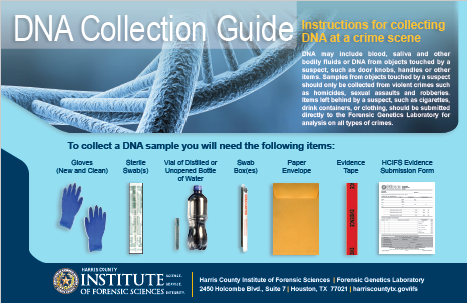The image is a low-quality infographic titled "DNA Collection Guide," created by the Institute of Forensic Science. The title is displayed prominently in the upper left corner in large white letters. The infographic uses colors like light blue, dark blue, gray, and red, with text in black and white. On the right side, there are detailed instructions for collecting DNA at a crime scene, emphasizing that DNA can include blood, saliva, and other bodily fluids, or be obtained from objects touched by a suspect, such as doorknobs and handles. These samples are particularly relevant in cases of violent crimes like homicides, sexual assaults, and robberies. Additionally, items left behind by a suspect, including cigarettes, drink containers, or clothing, should be sent directly to the Forensic Genetics Laboratory for analysis. 

Below the instructions is a recommendation for the necessary equipment to collect a DNA sample: gloves, sterile swabs, a vial of distilled or open bottle of water, swab boxes, paper envelopes, evidence tape, and evidence submission forms. There are illustrations accompanying these items, including a pair of gloves and other sample collection instruments and documentation. The infographic also features an amplified image of a DNA double helix, depicted like a spiraling ladder, to visually reinforce the focus on DNA evidence. The flyer ends with the Institute's contact information, and beige-yellow highlighted sections for critical instructions.